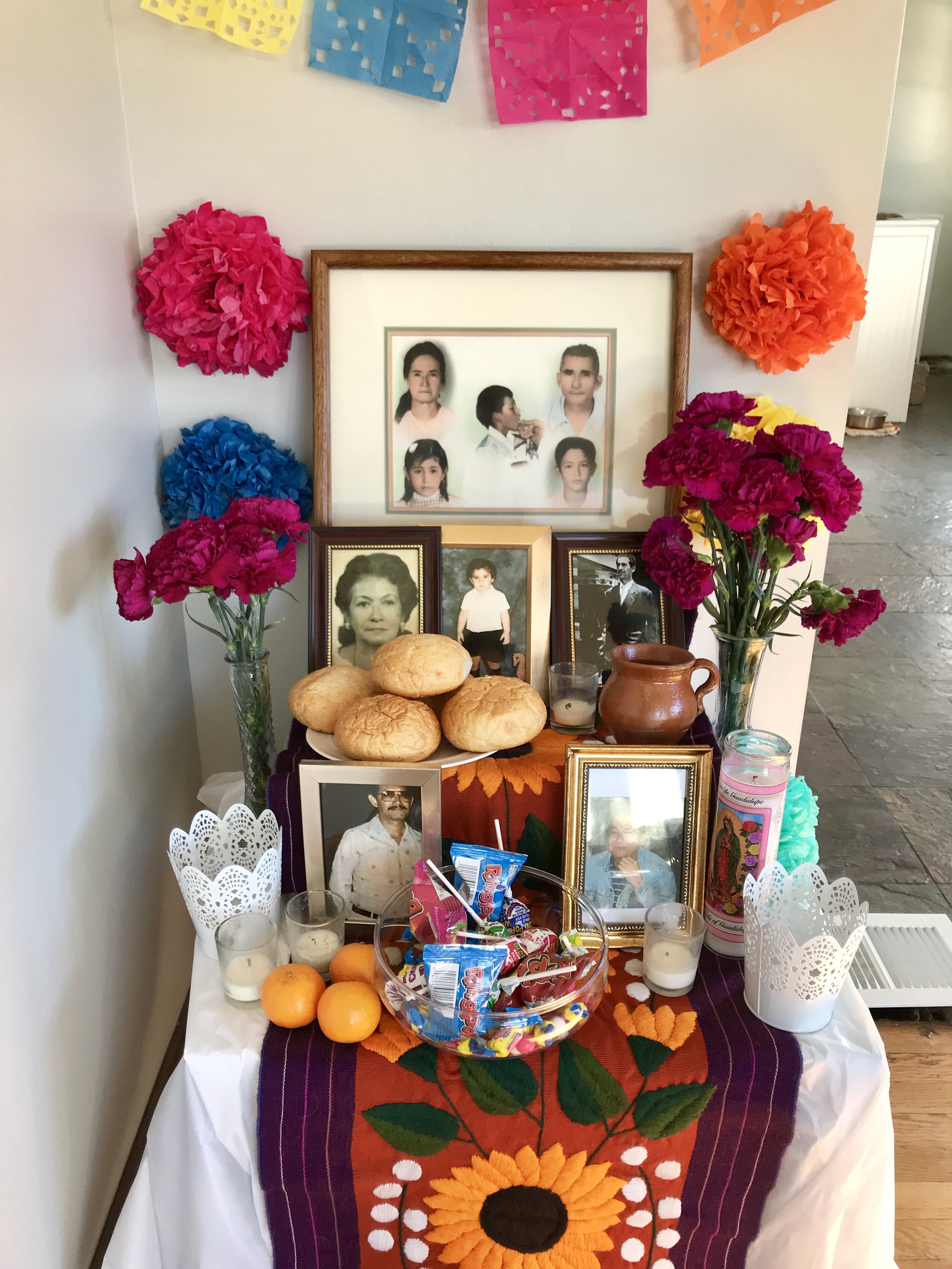The corner of the room is adorned with white walls, elegantly decorated with various embellishments. At the top, there is a decorative band featuring a series of colors—white, blue, pink, and orange—though it is partially obscured. Beneath this band, the walls are adorned with beautifully arranged flowers in a descending color order: pink, blue, orange, and yellow. 

A collection of picture frames, each holding cherished photographs, is displayed on the walls. The frames vary in color, with some being brown and others gold, and contain images of different people. One frame features a single female, another displays a single male, and yet another captures the essence of a family moment, showcasing a male and female with three children.

Below this display, a table holds a small assortment of items. Three oranges are neatly arranged alongside a bowl filled with various candies, including Ring Pops. A set of white candles stands beside the bowl, adding a serene ambiance. Additionally, a clear vase filled with vibrant pink flowers further decorates the table, contributing to what appears to be a thoughtfully assembled altar-like area.